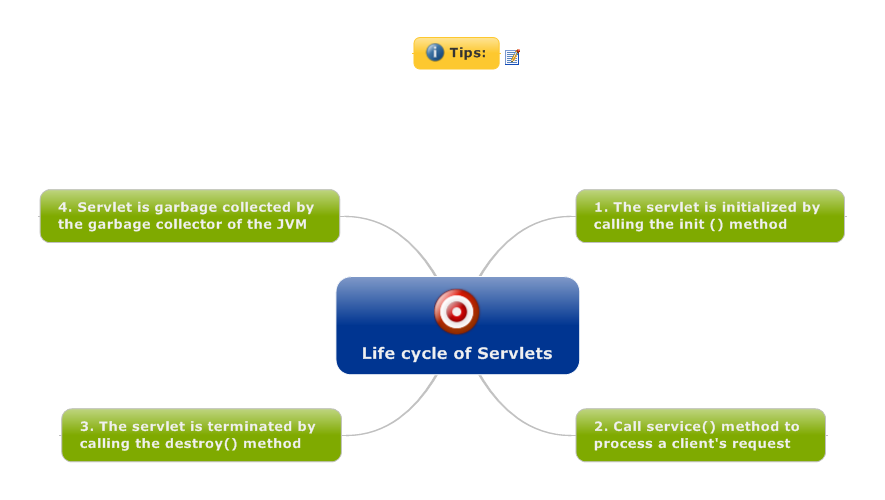The image is a detailed chart illustrating the life cycle of servlets, prominently featuring different colored text boxes against a plain white background. At the top, there's a yellow text box with black text that reads "Tips," accompanied by a small icon of a paper and pencil. Centrally located is a large blue rounded rectangle, containing the white text "Life Cycle of Servlets" and a red and white target-like icon. This blue box is connected by four curved lines to four green rounded rectangles, each outlining a different step in the servlet life cycle in white sans serif font. The steps, from top left and moving clockwise, include: "The servlet is initialized by calling the init method," "Call service method to process a client's request," "The servlet is terminated by calling the destroy method," and "The servlet is garbage collected by the garbage collector of the JVM."